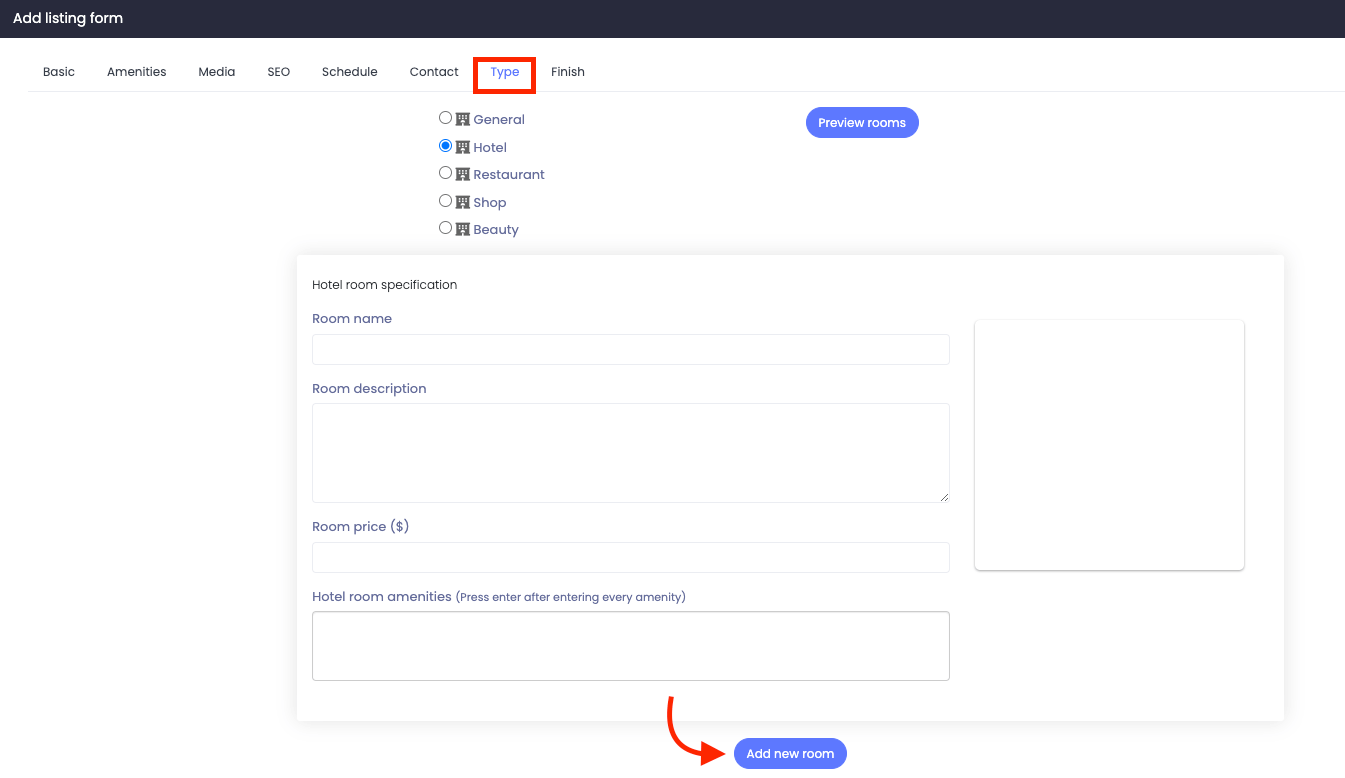This horizontal image appears to be a screenshot from a computer interface, specifically an "Add Listing Form" page for hotels or similar establishments. The form features a clean, white background with a top border that runs horizontally across the screen. On the left-hand side of this border, the text "Add Listing Form" is displayed in white.

Below the top border, there are several category tabs in black, all capitalized: "BASIC," "AMENITIES," "MEDIA," "SEO," "SCHEDULE," and "CONTACT." One of the categories, "TYPE," is highlighted in turquoise and enclosed in a red rectangle, indicating it is the selected tab. The "FINISH" category is listed in black.

Under the "TYPE" tab, a list of options appears, each with a circular selection box in front. The options are: "General," "Hotel" (this one is selected, with a turquoise dot in the circle), "Restaurant," "Shop," and "Beauty." To the right of this list, there is a blue, horizontally-oriented oval button with white text that reads "Preview Rooms."

At the bottom of the image, another white rectangular section is displayed, containing fields for "Hotel Room Specification." These fields include "Room Name" with an empty text box, "Room Description" with a larger empty rectangle for text input, "Room Price," and "Hotel Room Amenities." Below the "Hotel Room Amenities" section, there is a red arrow pointing downwards and another blue oval button with white text that reads "Add New Room."